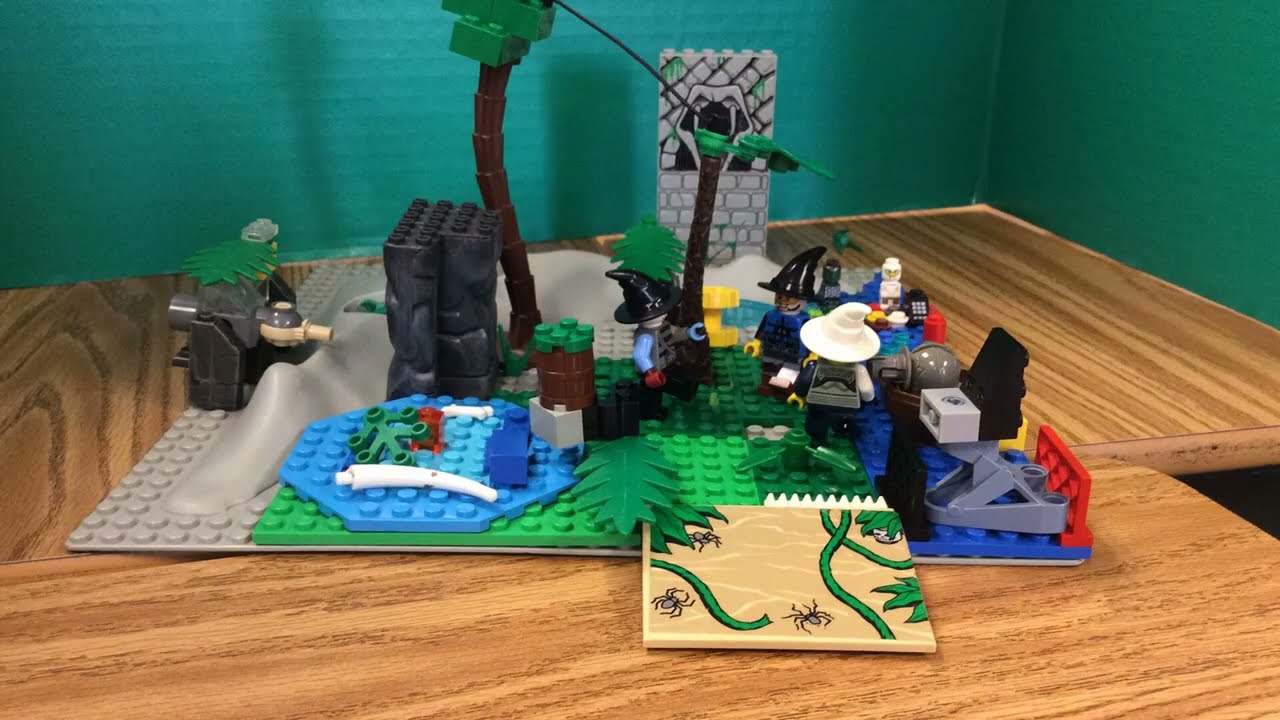In the image, we see a meticulously crafted Lego display set atop a wooden table, reminiscent of a child's work. The scene is structured to resemble a bustling tropical city, complete with detailed pavements, roads, lakes, trees, and various Lego people. The Lego figures are adorned with a variety of hats and helmets, creating a lively diorama. To the right, blue Lego pieces depict water, suggesting a lake or coastal area, complete with palm trees. To the left, a puddle and a tall rock add to the natural landscape. The intricate arrangement includes sand-like areas and grassy patches, contributing to the tropical island theme. Behind the table, a green wall provides a contrasting backdrop, highlighting the vibrant colors of the Lego city. There are no other people visible in the photograph, keeping the focus squarely on the elaborate Lego creation.